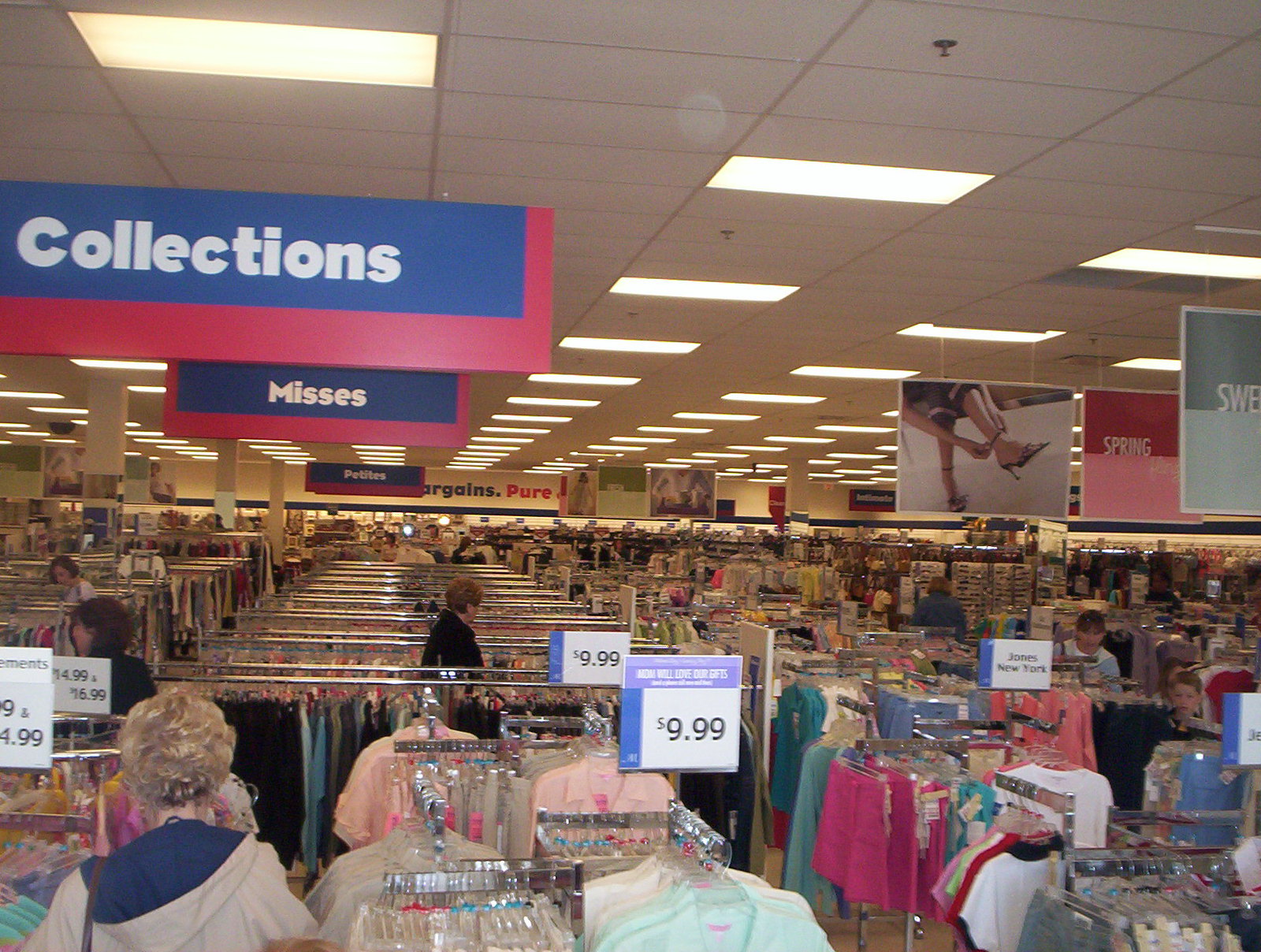In the detailed image, we see the bustling interior of a large clothing store, characterized by rows and rows of garments displayed on metal racks. In the foreground, a shopper with very short hair, dressed in a gray sweatshirt with a blue hood, is seen from behind. Various shirts, predominantly light blue and pink, hang on the racks with prominent price signs reading $9.99 in black text, while other signs in the distance show prices such as $14.99 and $16.99. 

To the right, a branded sign for "Jones New York" is visible, surrounded by more clothing items. The store appears vast, with numerous aisles extending into the distance, giving the impression of a significant retail space. Overhead, large aisle signs include sections like "Collections" on a dark blue and red background, and another labeled "Mrs." An additional segment is indicated, likely saying "Petites," although partially obscured.

The ceiling, composed of gray tiles and illuminated by rectangular beams of fluorescent lights, casts an even glow throughout the store. Along the upper walls, which are painted a light yellow, there's partial blue lettering and the word "pure" in red. The demographic of shoppers appears to be mostly older Caucasians, with a mix of women, a young boy, a young girl, and other indistinct figures, all engaging with the store’s extensive offerings.